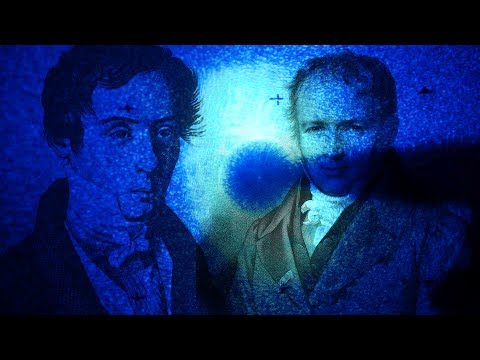The image depicts two men standing against a vivid blue, speckled background with black rectangular bars at the top and bottom. The scene has a gothic, almost Victorian feel, reminiscent of Edgar Allan Poe-era portraits. The man on the left, partially obscured by a blue cloud with white speckles, has fuzzy black hair and is staring slightly to the right. He wears what appears to be a suit with a necktie. The man on the right, whose face is brightened by a bright green sphere in the background, also sports a suit and has a receding hairline. He seems to be smiling ever so slightly while looking forward. A notable feature is a large circular disc with a hollow center located in the middle of the image, adding to the mysterious ambiance. The entire image seems grainy and almost otherworldly, like a scene from a painting or an old film.